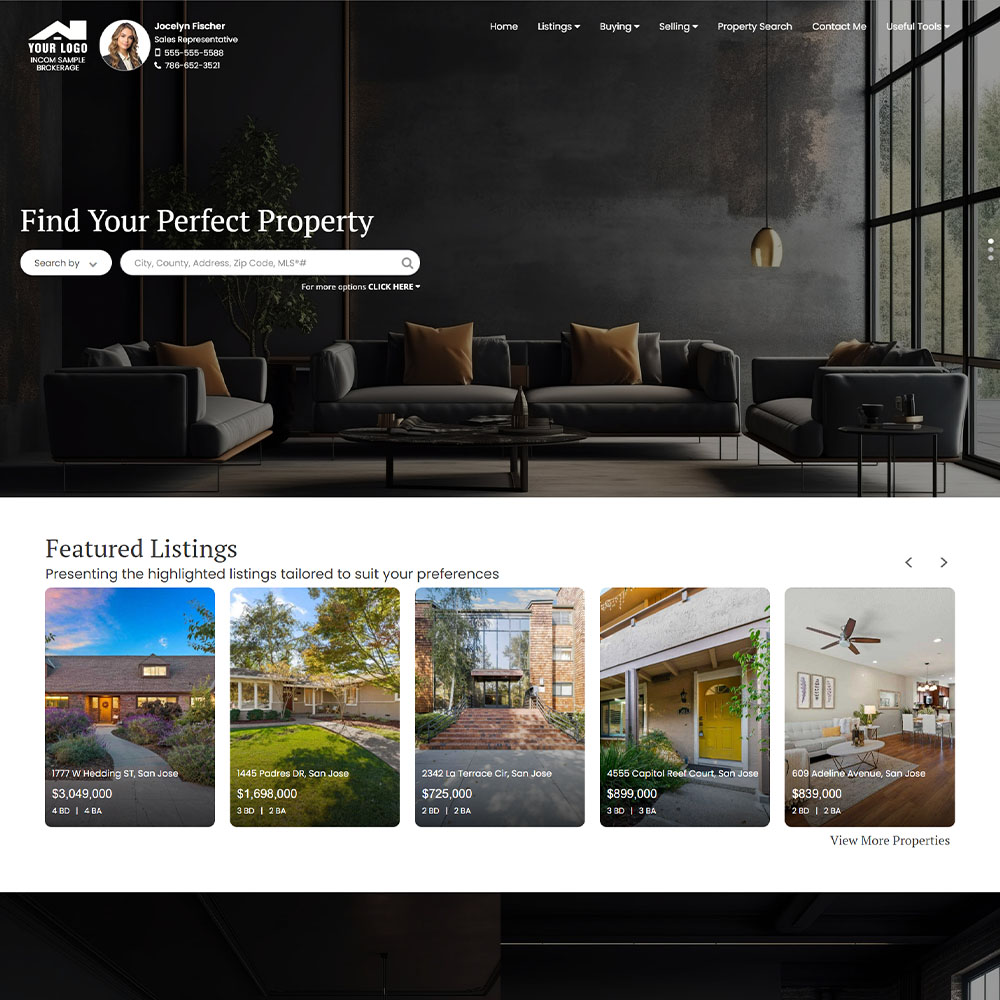This screenshot captures a comprehensive overview of a real estate brokerage website. The header prominently displays the company's logo alongside contact information for Jocelyn Fisher, a sales representative, including two phone numbers.

The navigation bar at the top offers various sections: Home Listings, Buying, Selling, Property Search, Contact Me, and Useful Tools. The main content area features a call-to-action banner titled "Find Your Perfect Property," accompanied by a search function allowing users to input criteria such as city, county, address, or zip code to refine their property search. Additional search options and a navigation indicator with three dots suggest the presence of multiple pages.

Further down, the website showcases its Featured Listings, presenting a curated selection of properties tailored to different preferences. Highlights include:

1. A luxurious four-bedroom, four-bath home listed at $3,000,000.
2. A spacious three-bedroom, two-bath property priced at $1,698,000.
3. A more affordable two-bedroom, two-bath residence for $725,000.
4. A three-bedroom, three-bath home available for $899,000.
5. Another two-bedroom, two-bath option listed at $839,000.

Each listing includes the property's address and a photograph. Users are also given the option to view more properties if they wish to explore additional listings.